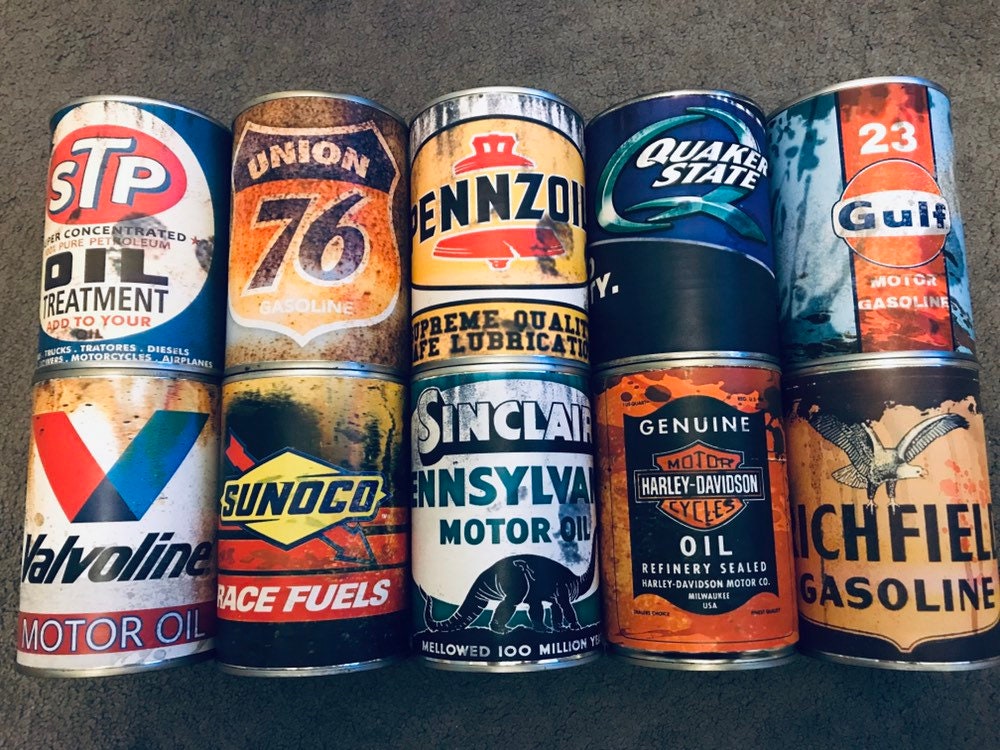The image depicts two stacked rows of vintage motor oil cans, totaling 10 items, set against a gray background. The top row features, from left to right, cans of STP oil treatment, Union 76 gasoline, Pennzoil motor oil, Quaker State oil, and Gulf 23 motor gasoline. The bottom row includes Valvoline motor oil, Sunoco race fuels, Sinclair Pennsylvania motor oil, Genuine Harley-Davidson motorcycles oil (refinery sealed), and an unidentified can with a logo featuring a bald eagle. Some of the cans appear to have oil streaks running down their surfaces, highlighting their aged and antique nature.